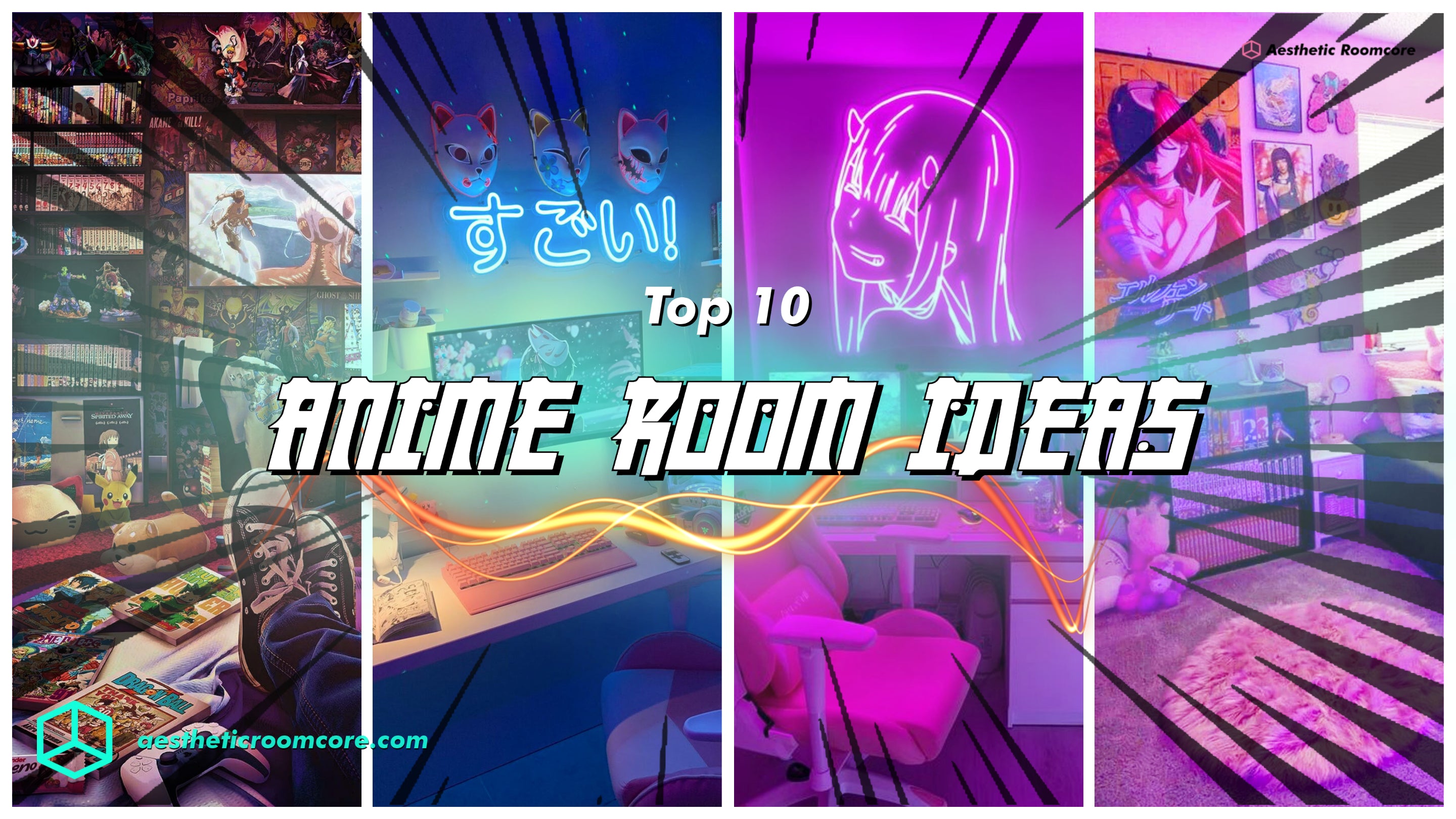The image is a collage of four vertical panels, each depicting different anime-themed rooms. Overlaid in large white letters in the center, it reads "Top 10 Anime Room Ideas." The four panels show varied room setups: 

1. The far left panel features a scene from the perspective of someone in a room, with their feet up, black and white shoes visible, facing a TV. The room is filled with various memorabilia, figurines, bookshelves, and Pokémon-themed items.

2. The next panel illustrates a computer station with a flat screen on a white desk, a keyboard, and a blue neon sign above it. The scene also includes three cat masks hanging on the wall.

3. The third panel reveals a pink-themed room with a pink desk and chair, and a pink neon image of an anime girl looking back over her shoulder.

4. The far right panel showcases another pink room adorned with several posters of women and movies, a low bookshelf filled with books, a pink area rug, and a bed.

At the bottom left corner of the image, there is a cube logo, accompanied by the website name "aestheticroomcore.com." A faint vignette effect with black lines draws attention towards the center of the collage.